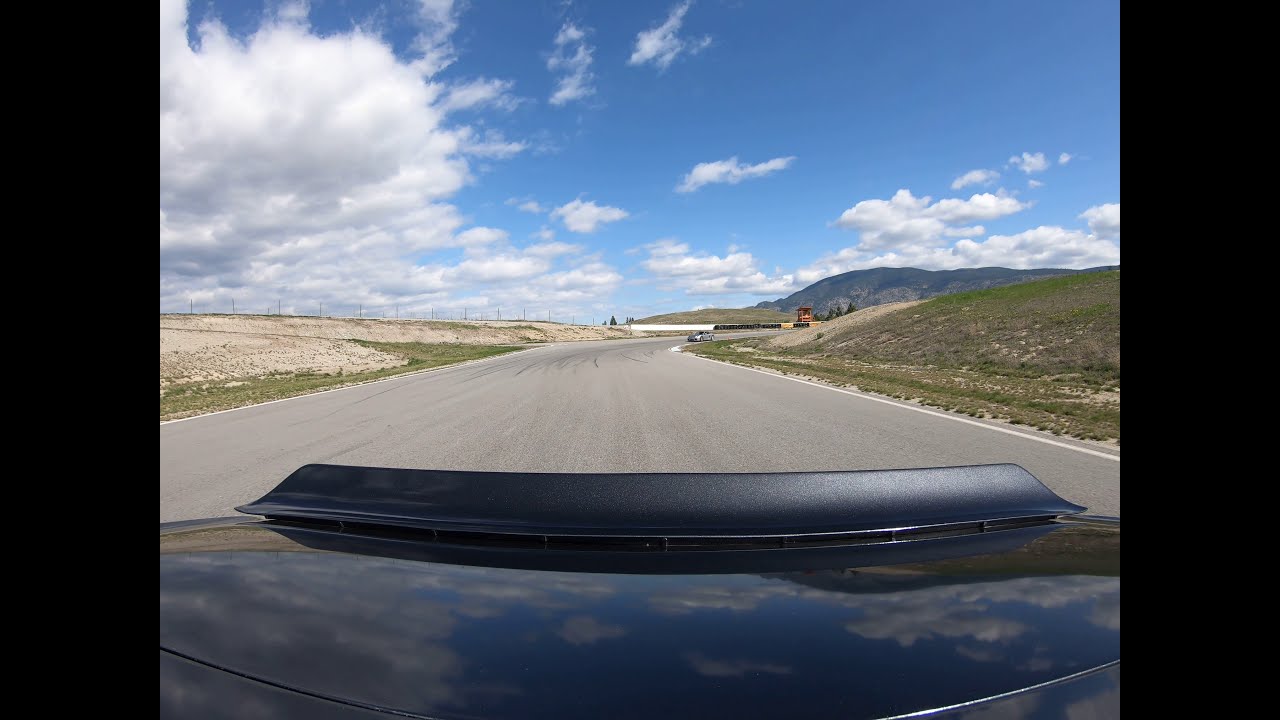This wide rectangular photograph, bordered by thick black rectangles on the left and right, appears to be taken from the rear window of a car. The glossy surface at the bottom, which reflects the sky, hints at the car's dark, perhaps blue or black color. A defining feature is the black spoiler on the back of this performance car, which suggests it might be on a racetrack.

The road extending into the horizon is gray asphalt with solid white stripes along its edges, devoid of any other markings, reinforcing the track-like appearance. The landscape to either side of the road is a mix of green grass, dirt, and sand, with a more mountainous terrain to the right and flatter land to the left. The road visibly curves to the right in the middle of the image.

In the distance, you can spot another small car, further supporting the impression of a racetrack setting. The sky, covering the upper half of the image, is a mix of blue and white with thick, fluffy clouds.absch